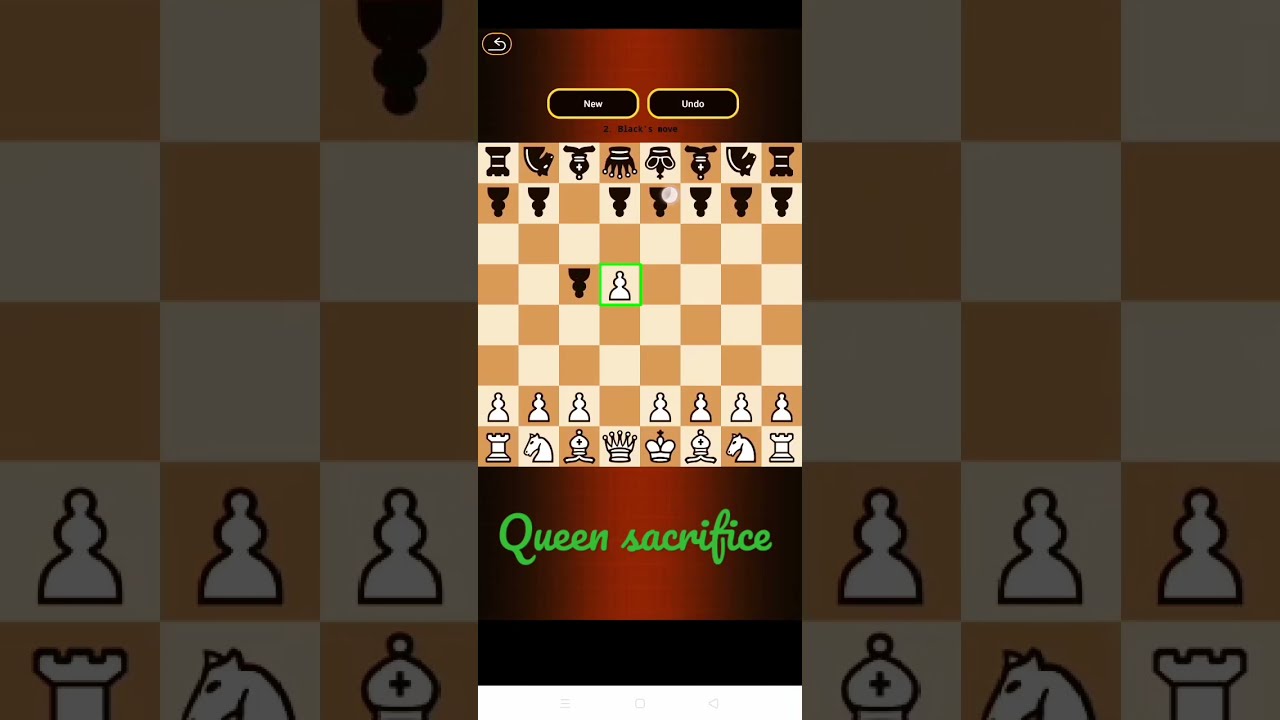The image depicts a mobile app screenshot of a chess game displayed in portrait mode with three distinct panels. The left and right panels show a slightly translucent, darkly lit chessboard with brownish-gold and white squares, featuring greyed-out chess pieces in the front six spaces, including pawns and other pieces. In the center panel, a brightly lit chessboard is shown in full view, highlighting an ongoing game. The board is divided with white pieces at the bottom and black pieces at the top. Notably, a white queen is positioned next to a black pawn in the middle of the board, emphasizing a pivotal moment in the game. At the bottom of the central panel, green cursive text reads "Queen sacrifice," indicating the move being described. The top of the screen displays a "New" button, an "Undo" button, and a back button in the upper left corner, suggesting interactive elements of the app. The background above and below the board is a shiny dark brown, framing the visual elements.